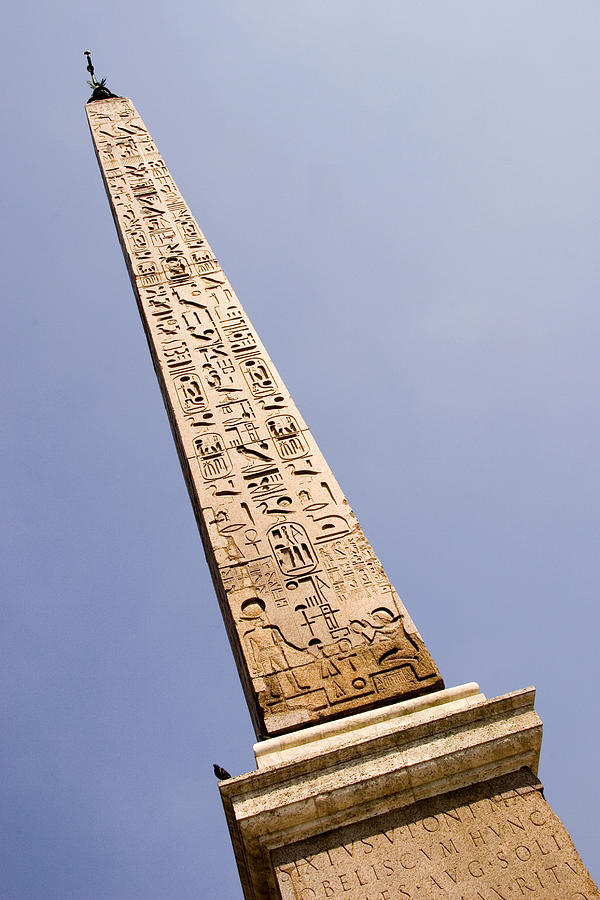The photograph captures a very tall, thin obelisk-like monument extending up to a striking height, possibly around 100 feet. The image is taken from the base, with the monument angled from the lower right to the upper left. The stone structure is predominantly a medium brown in color and tapers to a pointed top, where a barely discernible metal spire comes into view. The foundation of the obelisk features carved text, likely in Latin, and the entire surface is adorned with intricate engravings, reminiscent of ancient Egyptian hieroglyphics, though not necessarily authentic. These carvings include a diverse array of figures, such as adults, children holding hands, birds, circles, eyes, and various dots, etched meticulously into the stone. In the lower part of the photograph, a small shelf with a bird perched on it can be seen. The backdrop showcases a clear blue sky with no clouds, enhancing the monument's imposing presence and detailed artistry.